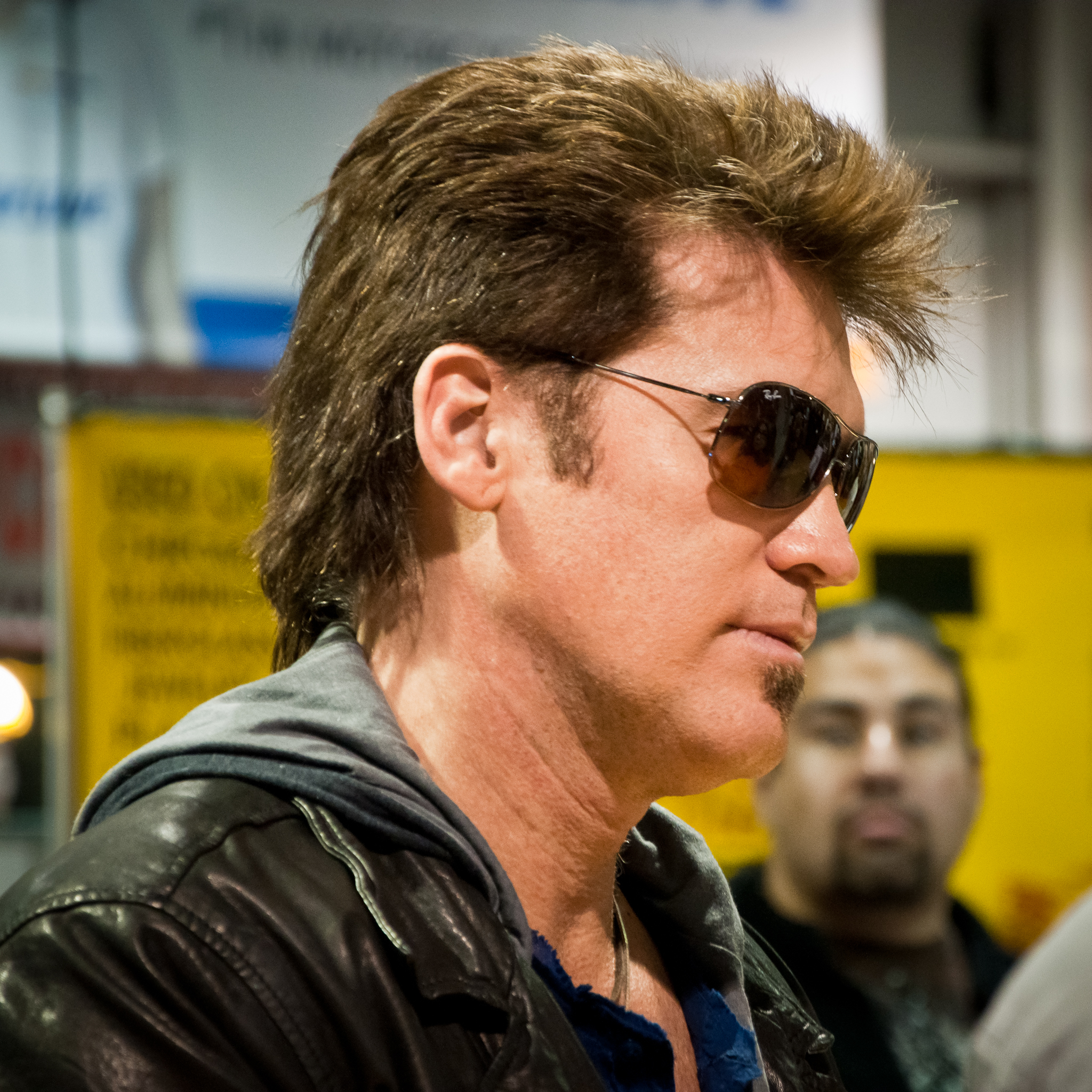The photograph captures a three-quarter profile of a man, possibly resembling musician and actor Billy Ray Cyrus, gazing towards the right. The man sports short, spiky dark blond hair with sideburns and a small goatee under his chin. He wears thin-framed black sunglasses with brown reflective lenses that obscure his eyes. His attire consists of a black leather jacket layered over a gray hoodie and a blue shirt. A gold necklace is visible around his neck. 

In the background, there is another man, blurred out, with a goatee and black hair. A yellow banner with indistinguishable black text on metal poles can also be seen, though it is out of focus. Further back, a large white wall completes the backdrop, suggesting the setting might be indoors.